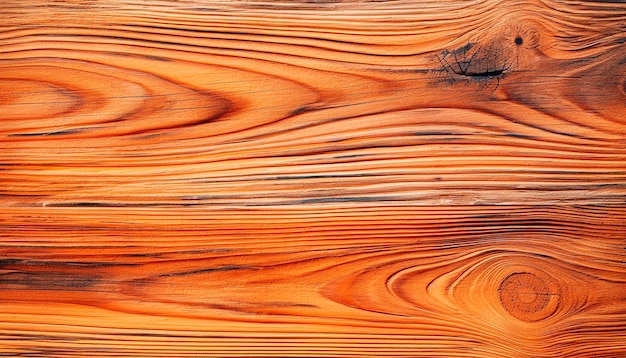This indoor close-up photograph captures the intricate details of a piece of wood, showcasing its distinct grain patterns and warm tones. The wood panel is cut flat, revealing a beautifully prominent and finished texture that might have been stained with oil. The overall coloration is a rich brownish-orange with subtle hints of gray running through the center. 

Dominating the scene are various sections of natural wood characteristics: in the lower right corner, a prominent knot with concentric circles radiates from dark brown to light brown, compressing the otherwise horizontal striations. Similarly, another knot is visible in the upper right corner, accompanied by darker and lighter bands and a noticeable crack that adds to the character of the wood. Around these knots, the darker rings are more compressed, starkly contrasted against the more evenly spaced lines running along the length of the wood. 

The panel also features additional swirls and wavy patterns, enhancing the natural beauty of the wood. These details attest to the organic complexity and visual appeal of the wood grain, making the entire piece an exquisite subject for close-up photography.